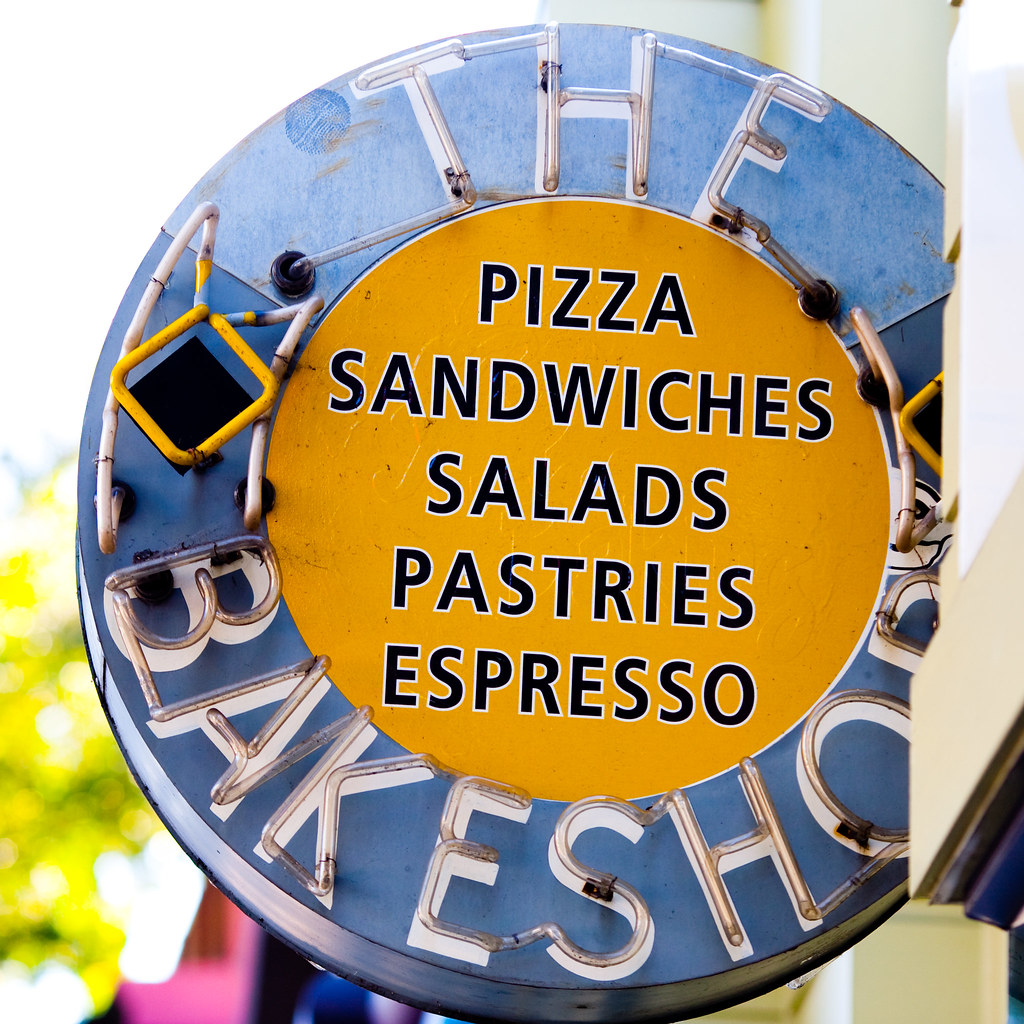This image depicts a circular storefront sign with a white background and a blue border, partially obstructed by a white building on the right. The top of the blue border features the word "The," and the bottom appears to read "Bake Shop," though part of it is cut off. Inside the blue-bordered circle, there's a golden yellow medallion with dark blue text arranged in five lines, listing the items available: "Pizzas," "Sandwiches," "Salads," "Pastries," and "Espresso." To the left of the sign, a blue tree can be seen. In the background, there are some elements of a greenish-pink hue, possibly from the environment around the sign, which itself appears to be mounted on a wall.